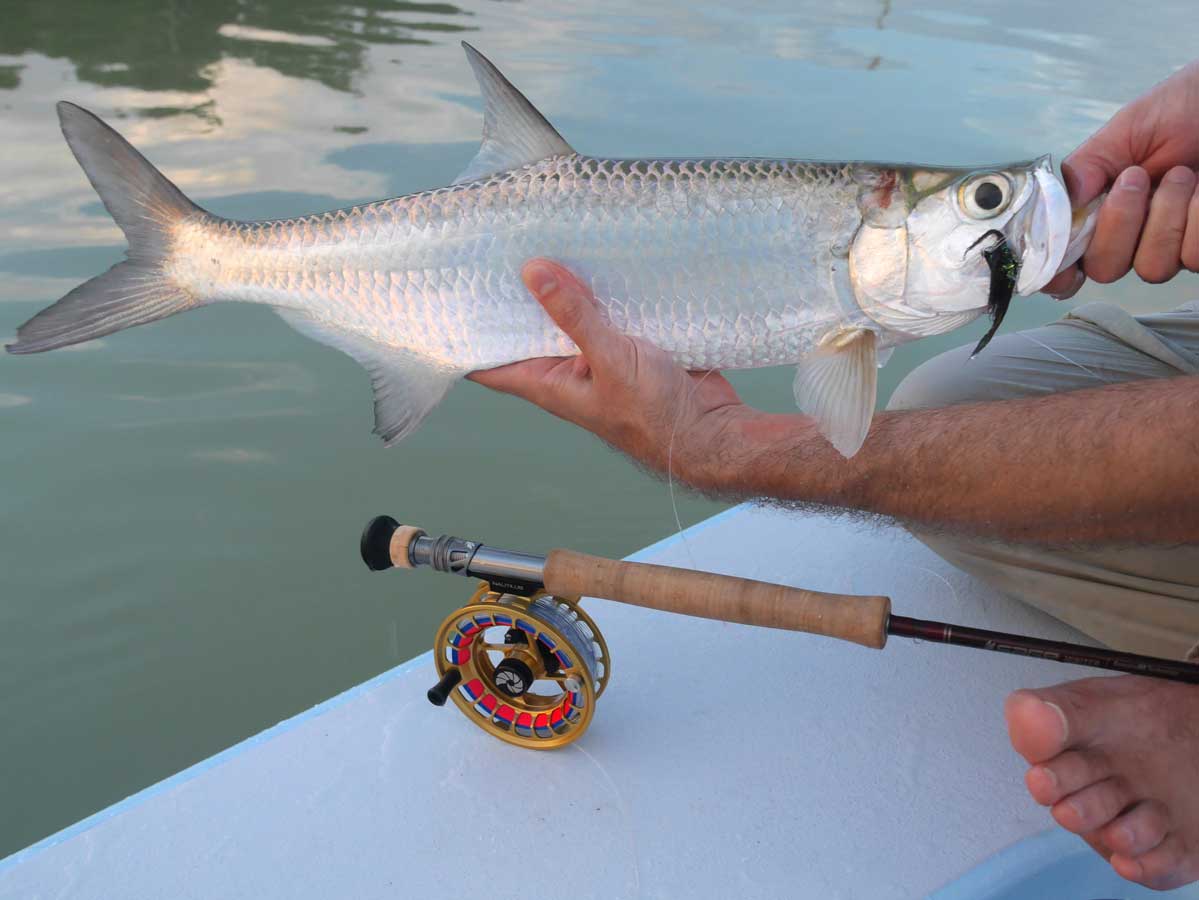In this horizontally aligned rectangular image, slightly wider than it is tall, a fisherman is prominently featured holding a gleaming silver fish against the backdrop of a calm, flat body of water. The fish, which is around 2 to 3 feet long, has a shiny body with textured irregular circle-like patterns and a gray tail and fins. Its large black eyes are notable. The angler's left arm extends from the right side of the picture, holding the fish with its head on the right and its tail on the left. His right hand is seen removing a hook from the mouth of the fish.

The top half of the image captures the serene water, while the bottom half shows the edge of a white boat extending from the upper right to the lower left. Visible parts of the fisherman include his right knee, left foot, left arm, and right hand. In the lower right corner, his toes are seen peeking from the boat.

A fly fishing rod, identified by its distinctive features, is present in the scene, with a grey reel, a black rod, and a brown cork handle. The rod’s position suggests it's being handled with the butt end to the left and the tip to the right. The dominant colors in this evocative image include shades of silver, brown, grey, blue, and beige.